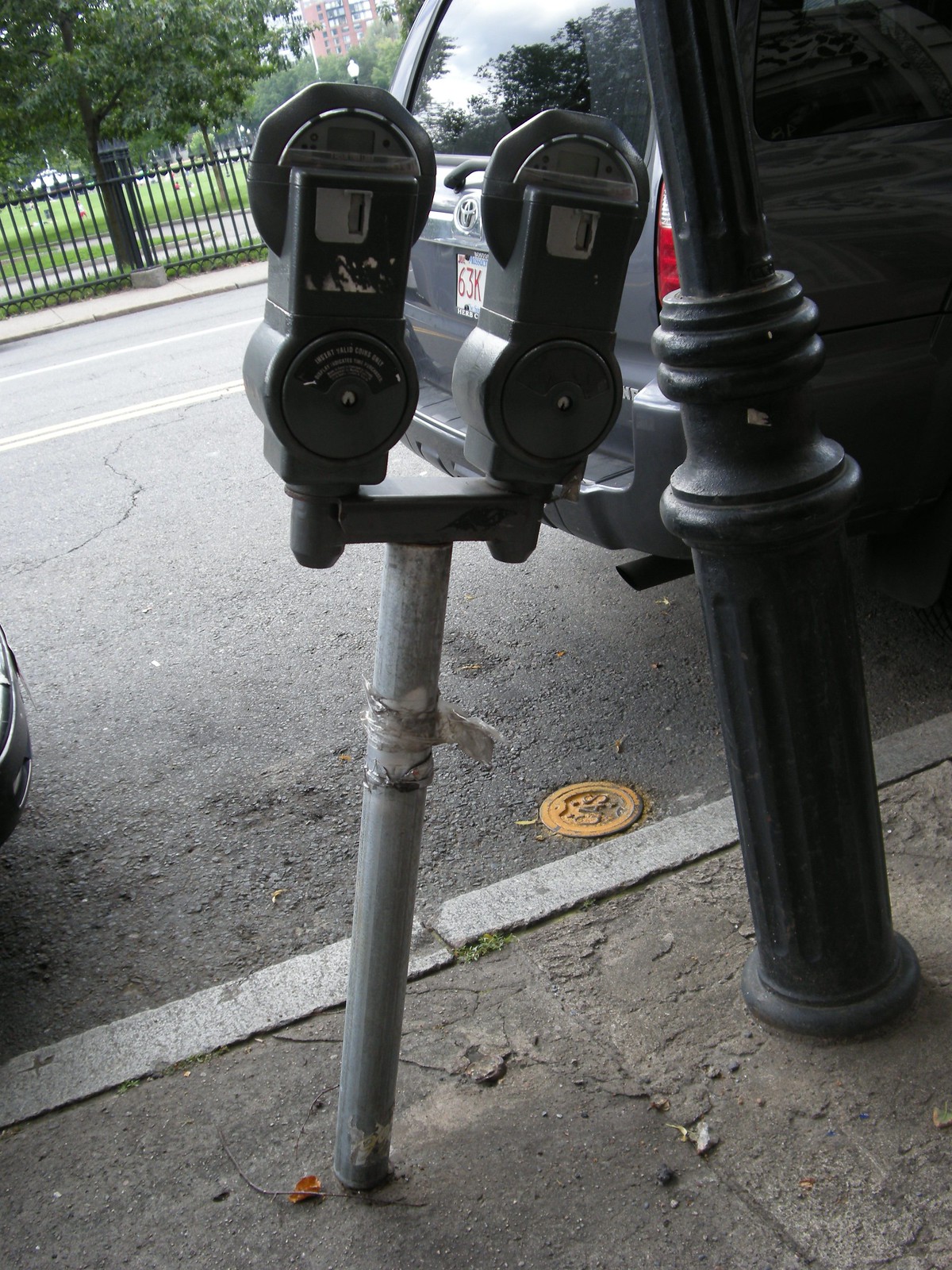This detailed photograph captures the scene of an old and weathered parking meter that dominates the frame, noticeably slanted at a 30-degree angle as though impacted by a collision. The parking meter, composed of a metallic pole leading to a weather-beaten, black pewter dual-meter unit, stands precariously on a concrete sidewalk that is nearly level with the adjacent street. To the right of the skewed parking meter, there is a meticulously engraved black pole, standing erect with a round base, adding contrast to the tilted meter.

The background features the rear of a Volkswagen SUV, identifiable by the partially visible license plate displaying "63K" in red. The scene also includes the faint appearance of another car's bumper to the left. The paved asphalt road, exhibiting signs of wear and minor cracks, separates the vehicles from a tall, black metallic fence that outlines a park area filled with greenery and a leafy tree.

Scattered twigs and leaves are present both on the sidewalk and the street, contributing to the slightly neglected atmosphere of the setting. The entire composition captures a snapshot of urban life, marked by elements of both decay and persistence.